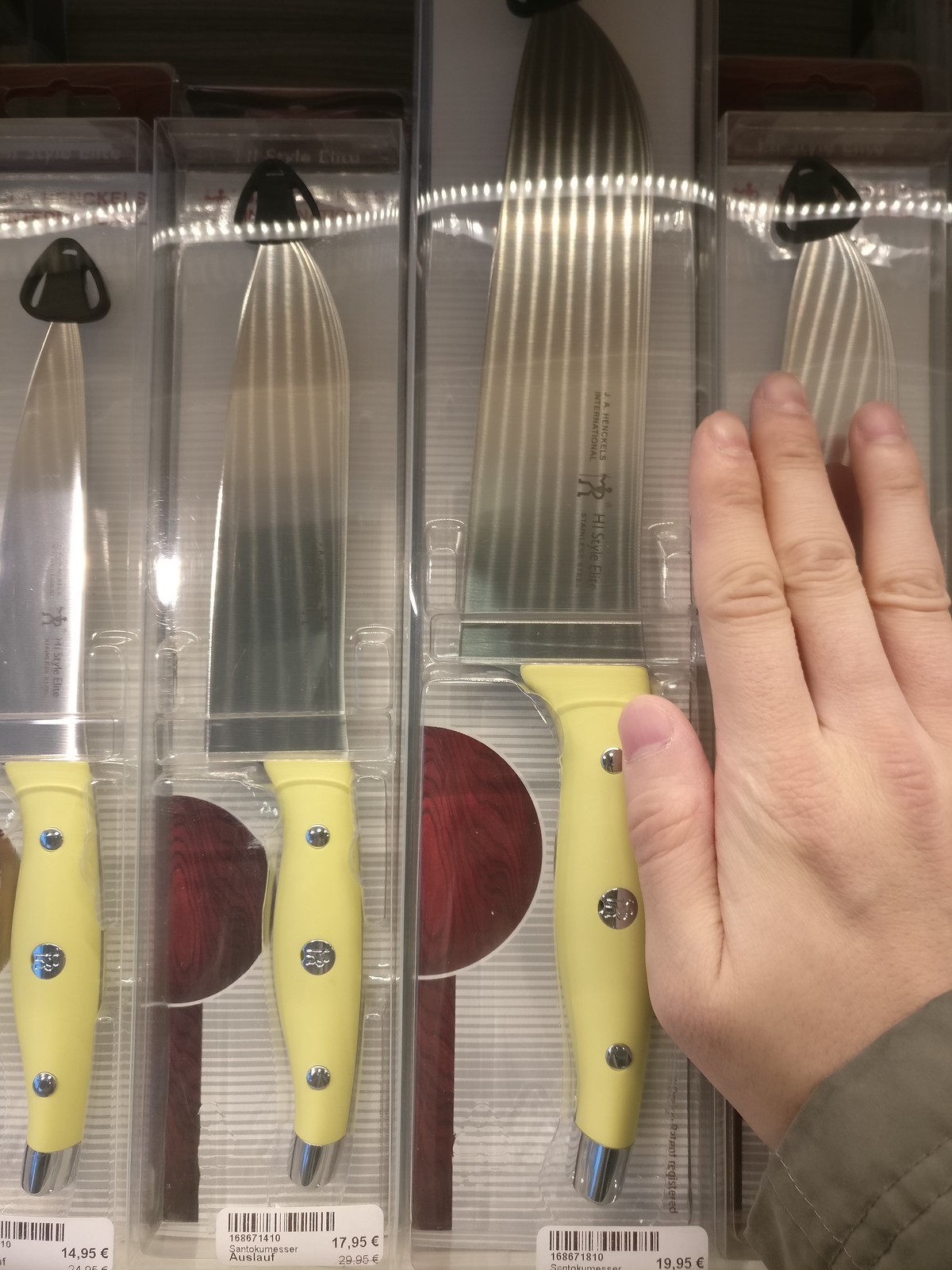This image depicts an assortment of packaged, brand-new knives displayed on store shelves. The knives share a consistent design, featuring yellow handles with chrome accents, including three distinctive silver circles on each handle. The blades themselves vary in shape, from rectangular to pointed, and exhibit some striped designs. The packaging indicates the knives are priced at 14.95, 17.95 (discounted from 29.95), and 19.95 euros. A left hand, partially seen with four fingers, clad in a thick grayish-green coat with decorative top stitching, is resting atop one of the packages, emphasizing the size comparison. The scene suggests the location could be in a European store, possibly Germany or Austria.